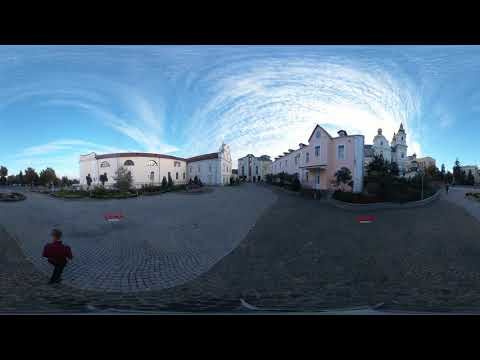The image depicts an outdoor scene with a slightly blurry and grainy quality, suggesting it was taken with a lower-tech camera. The main subject is a small figure on the left, possibly a child, wearing a red top and blue jeans, walking on what appears to be concrete or a sidewalk. The person is heading towards a cluster of houses or townhouses in the background, which exhibit the style of small European buildings or cottages. The area looks relatively quiet and desolate, with just a few other people visible in the distance. The sky, a light blue expanse, features a striking formation of wispy, swirling clouds that draw the eye. The scene also includes patches of grass, with some areas differing in color, adding an element of visual contrast. The overall impression is of a serene, somewhat isolated neighborhood, backdropped by an interesting sky and humble, yet quaint, structures.